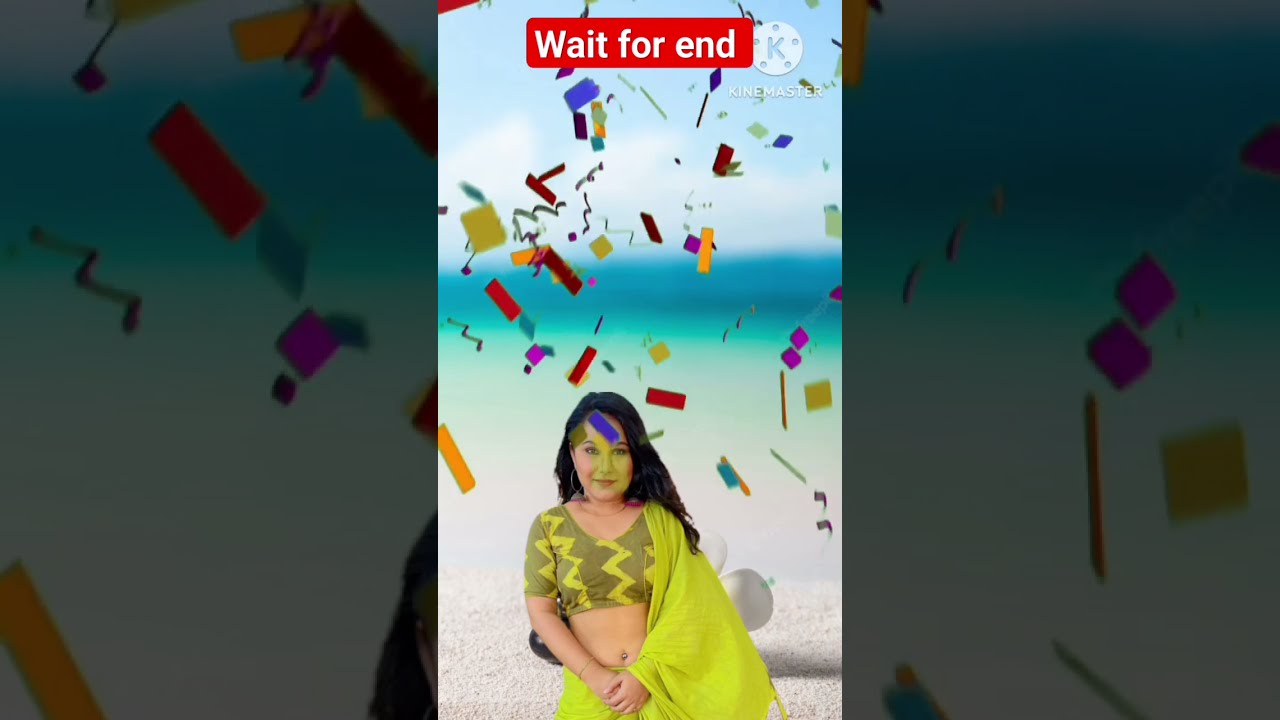In this photograph, a woman is captured on a beach, standing well forward of the shoreline with a blue sky and a turquoise and ultramarine sea blurred in the background. She appears to be in her late 30s or early 40s, and is dressed in a traditional bright yellow sari that drapes over her left shoulder, paired with a short sleeve midriff-baring blouse. A matching bright yellow skirt completes her attire. Her hair is down, and she has a slight, happy smile as she looks directly into the camera. Above her head, confetti and streamers are suspended in mid-air, suggesting a celebratory moment. The photo features a red bar with white lettering at the top that says "wait for end," and faintly in the top right-hand corner, the watermark of the video editing company "KineMaster" can be seen.